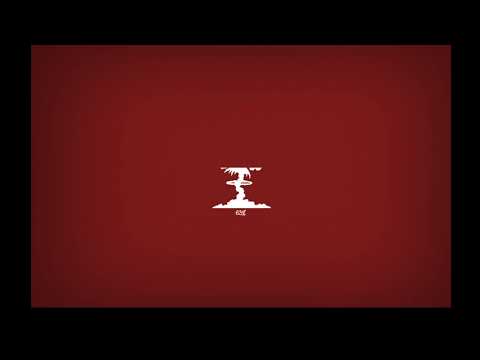The image depicts a square thumbnail with a thick black border surrounding a maroon rectangle that has a gradient fill, transitioning from a brighter red in the center to darker shades towards the edges. The upper right corner of the square is folded over, dog-ear style. Positioned in the center of the maroon rectangle is a complex white graphic. At first glance, this graphic resembles the bottom of a palm tree with a bendy trunk, but upon closer inspection, it could also be interpreted as the mushroom cloud of an atomic blast. The tree or cloud structure has a ring around its center, and there is an additional horizontal layer halfway down. Beneath this layer, it appears to form a mountain shape with tiny, illegible letters at the bottom. The upper left corner of the square contains a white circle set against a blue background, the lower left corner features something green, and the lower right corner displays a diagonal white bar extending from the bottom center to the middle right edge. This thumbnail icon is typically seen when an image has failed to load or is unavailable for viewing.